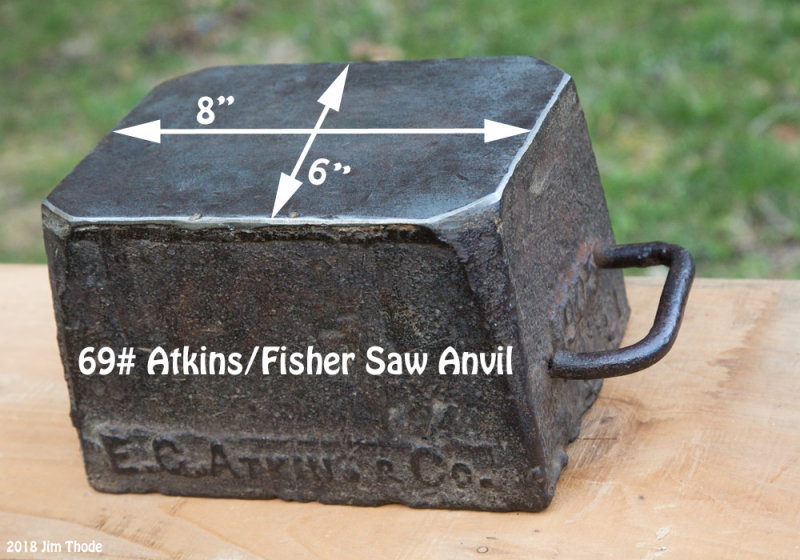The photograph depicts a robust, rectangular anvil made by E.C. Atkins and Company, resting outdoors on a wooden table against a blurred grassy background. The anvil, which is a solid block of metal with a handle protruding to the right, is engraved with "E.C. Atkin RCC" on the side, indicating its manufacturer, while additional digital text overlays it, reading "69 # Atkins/Fisher saw anvil." The clearly visible proportions of the top surface measure 8 inches by 6 inches. The image, attributed to Jim Thode and dated 2018, captures the anvil in bright outdoor light, emphasizing its substantial build and utilitarian purpose for metalworking tasks like straightening or hammering hard metal objects.